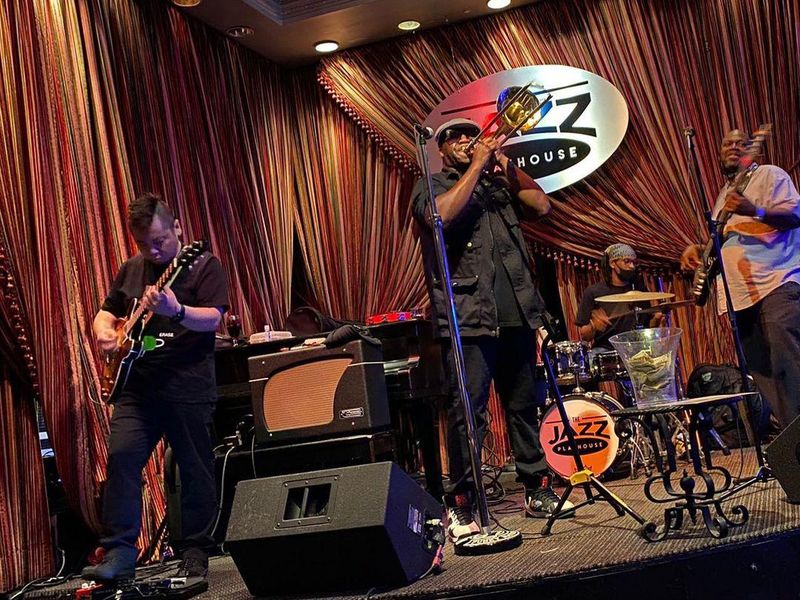This photograph captures a lively performance by a jazz band on a black rectangular stage adorned with a swagged and multi-shaded orange-striped curtain in the background. Situated amid recessed spotlights that cast a purple hue, the band consists of four men, each seemingly in their 20s or 30s. On the far left, an African American man is playing an electric guitar, flanked by various pieces of stage and sound equipment. Near him stands another man, identifiable by his sunglasses, skillfully playing a trumpet near a microphone. Toward the right side of the stage, an Asian band member handles a bass guitar, also positioned in front of a microphone. At the very back, the drummer, whose bass drum proudly displays "Jazz Playhouse," anchors the ensemble. There are a few amplifiers scattered across the stage and, importantly, a small table with a glass vase for audience tips, inviting support for the captivating musical experience.